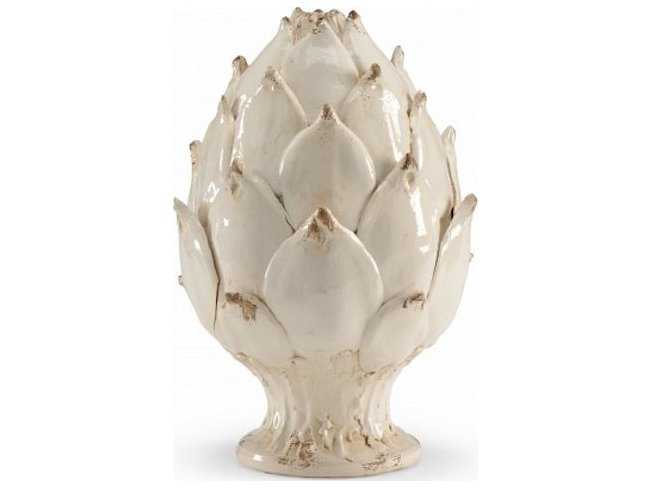The image depicts a ceramic figurine designed to resemble an artichoke, primarily cream-colored with some pinkish-brown tips. The figurine stands on a small pedestal and has a smooth, shiny glaze that reflects light. The textured surface and the bumpy base contrast with the sleek leaves that point upwards. Slight scuff marks on the bottom and leaf tips contribute to its vintage, antique appearance, suggesting it could be a handcrafted piece from a pottery or ceramics class. The overall look is reminiscent of a delicate, collectible item you might find in an antique shop.